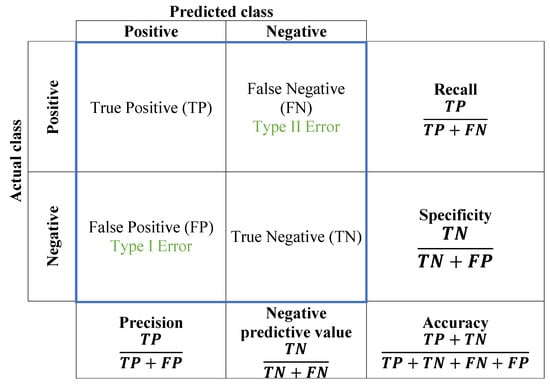The image is a detailed infographic chart depicting classification metrics and error types for a predictive model. 

At the top and left side, it categorizes data into 'Predicted Class' and 'Actual Class' with labels for 'Positive' and 'Negative' in black text. The chart includes four main boxes bordered in blue: 'True Positive (TP)' and 'False Negative (FN)' on the top row, and 'False Positive (FP)' labeled with a Type 1 error indication, and 'True Negative (TN)' on the bottom row. 

Each section provides specific performance metrics: 
- 'Precision' (TP / (TP + FP)), indicating the accuracy of positive predictions.
- 'Negative Predictive Value' (TN / (TN + FN)), showing the proportion of correct negative predictions.
- 'Recall' (TP / (TP + FN)), reflecting the true positive rate.
- 'Specificity' (TN / (TN + FP)), representing the true negative rate.
- 'Accuracy' (TP + TN) / (TP + TN + FN + FP)), measuring overall classification performance.

All elements are drawn with black lines, and the text within the boxes is also black, emphasizing the various metrics and their formulas clearly. The diagram systematically outlines the relationship between prediction outcomes and actual outcomes, while distinctly highlighting the roles of true and false positives and negatives.